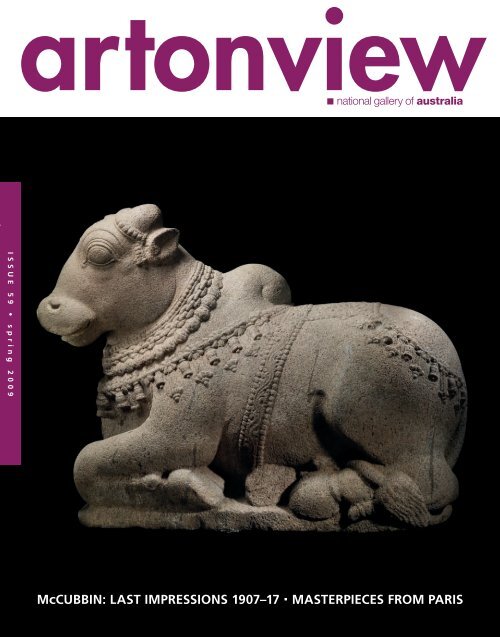This is a scan of a magazine cover, prominently featuring "Art in View, National Gallery of Australia" in a purple font against a white background at the top. Beneath this, taking up the majority of the image, is a black background showcasing a sculpture of a cow. The sculpture, which appears dark gray and fashioned from rock, is depicted lying down with its hooves tucked underneath it and facing towards the left. The cow has a blanket draped over its back. Below the cow, the white text reads, "McCubbin, Last Impressions, 1907-17, Masterpieces from Paris." On the left side, a purple box matching the title font contains vertically-aligned white text stating, "Overton View, Issue 59, Spring 2009."